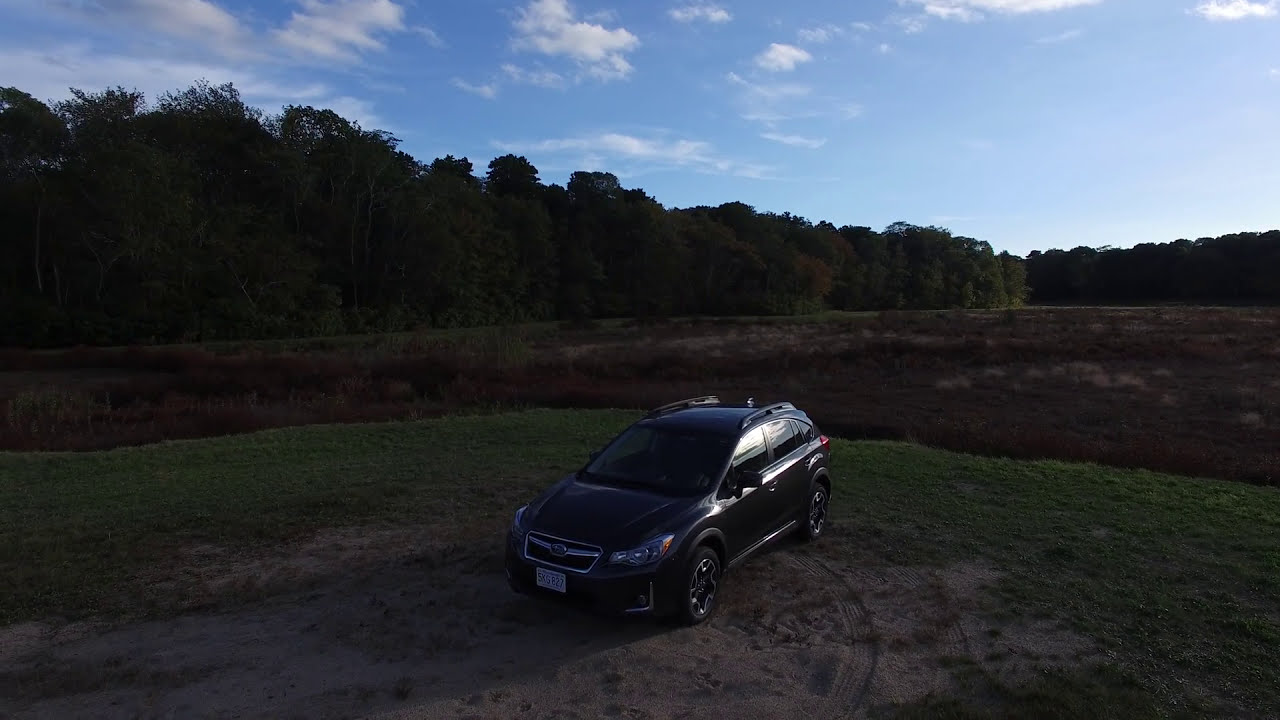The image depicts a secluded outdoor area under a vibrant, blue sky with scattered white clouds, prominently towards the left. Dominating the background is a dense line of tall, green trees, characteristic of a forested region. In front of this tree line, the ground transitions from a patchy brown dirt field to a mix of short green grass and bare earth in the foreground. Sitting centrally in this scene is a single black SUV with four doors and a distinctive hatchback shape, featuring an arched body and roof rails on both sides. The SUV has black tires and dark-tinted windows, with light reflecting off the right side windows. The front license plate, bearing the number "5KS827," is clearly visible, though the state or province isn't legible. The scene is devoid of any human presence, emphasizing the stillness and isolation of the location.